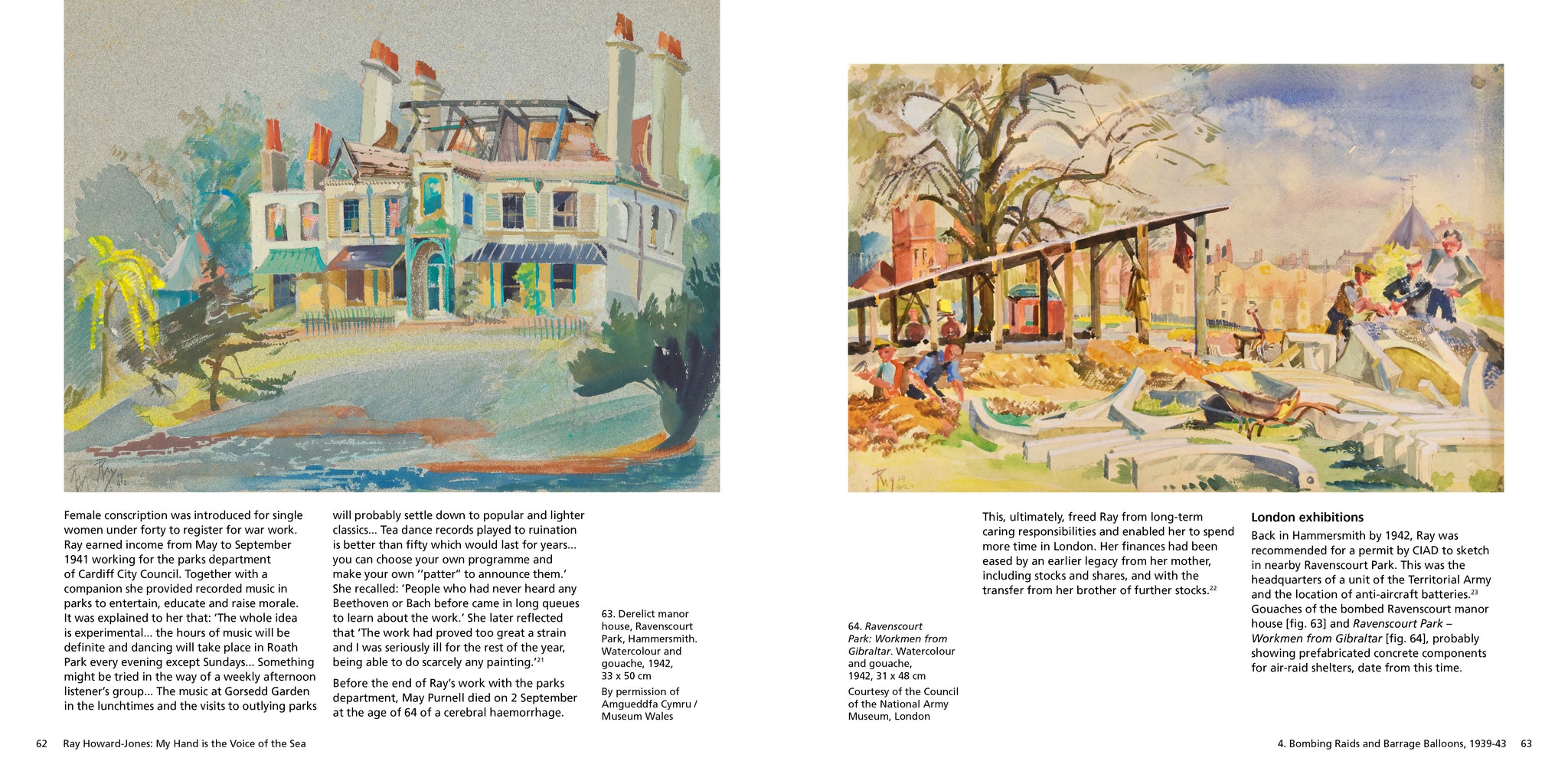The image depicts a two-page spread from a coffee table book featuring two distinct watercolor paintings by Ray Howard Jones. On the left, the painting titled "Derelict Manor House, Ravenscourt Park, 1942," showcases a semi-constructed white house with an array of wild, vibrant colors. The house has several chimneys, blue awnings, and numerous windows, surrounded by yellow and green foliage. The foreground features tropical plants, and the background is a colorful blur, indicating an unfinished state with only the foundation and red-topped steeples. Text at the bottom reads, "My hand is the voice of the sea" and details the painting's exhibition status and history.

On the right, another painting from the same era shows an outdoor scene with young men involved in a construction project. A ladder lies on the ground, and a wheelbarrow is centrally placed among the activity. The scene also includes a steeple in the distance and additional construction outlines, with a tree and vaguely colored buildings in the background. The colors in this painting include blue, white, pink, yellow, black, and gray, consistent with the watercolor style. Both paintings are described in detail with historical context relating to wartime activities in London exhibitions.